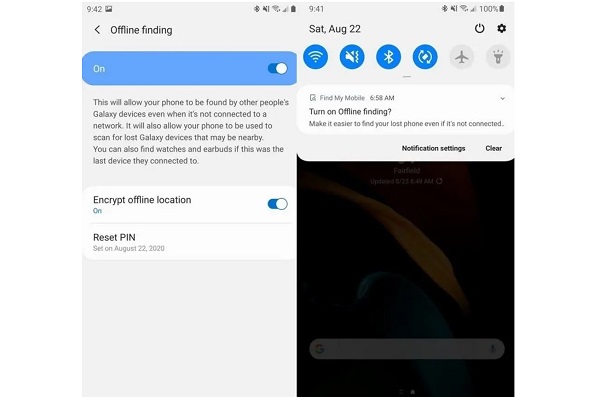The image is a side-by-side screenshot from a cell phone. The right side displays a "Find My Mobile" screen with the time 9:42 and the status "Offline finding." A blue switch labeled "On" indicates that offline finding is enabled, allowing the phone to be located by other Galaxy devices even when it's not connected to a network. Additionally, this setting enables the phone to scan for nearby lost Galaxy devices, including watches and earbuds, if they were last connected to this phone. Below this, on a white background, there's a setting for "Encrypt offline location," which is also turned on, shown by a blue switch with a white circle on the right. Further down, there's information about a reset PIN set on August 22nd, 2020.

The left side of the screenshot shows the phone's status bar with the time 9:41 and the date Saturday, August 22nd. Below the date, icons for Wi-Fi, sound, Bluetooth, and screen rotation appear in blue, while airplane mode and flashlight icons are gray, indicating they are off. The sound icon indicates the phone is set to vibrate mode. Underneath, a "Find My Mobile" notification from 6:58 a.m. advises the user to "Turn off offline finding" with a brief description: "Make it easier to find your lost phone even if it's not connected." There's an option for notification settings and a "Clear" button in black.

In the background, a faint glimpse of the home screen is visible, featuring a Google search bar at the bottom and what appears to be an abstract wallpaper with blue and yellow paint swirls. There is no additional text visible. The overall purpose of the image is to highlight settings related to finding a lost phone or other connected devices when they are offline.